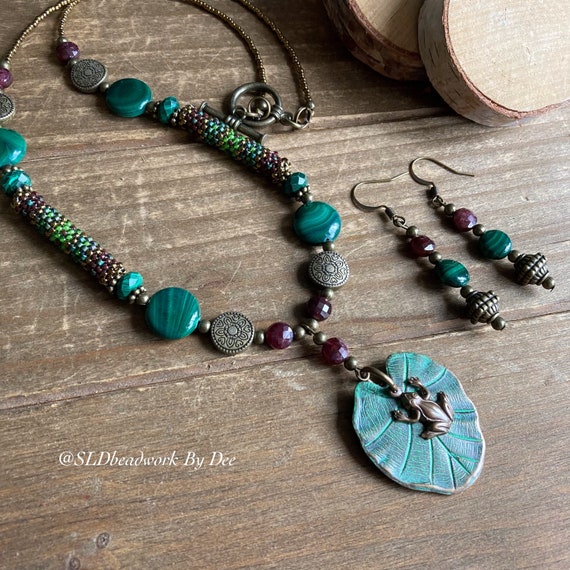This detailed photograph showcases a handmade set of bead jewelry consisting of a necklace and two dangling earrings. The set, created by the artist Dee, features a combination of deep purple and green beads. The necklace prominently includes a large pendant designed as a lily pad with a bronze frog at its center. Both the necklace and the earrings possess a cohesive design language, integrating similar dark blue, purple, and green beads along with intricate metalwork. The jewelry is artistically displayed flat on an unvarnished, rough-hewn wooden tabletop, adding a rustic charm to the image. Notably, the lower left corner of the photograph displays bold white italicized text that reads "@SLDBeadwork by Dee," directing viewers to the artist's website, sldbeadwork.com, for more information.